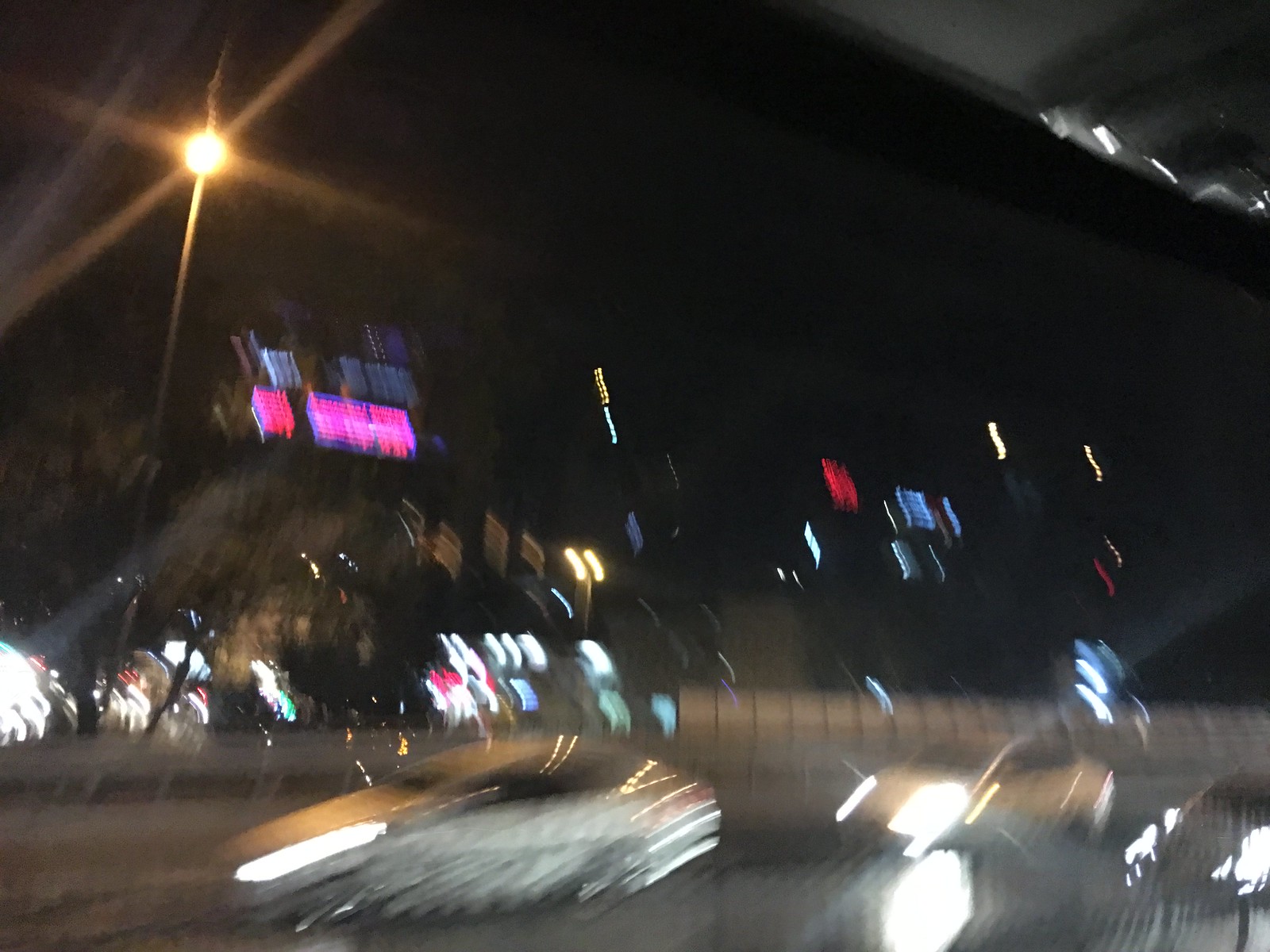This photograph captures an accidentally taken, very blurry night scene of a busy city street. Central to the image is a dimly visible roadway with two lanes of traffic, featuring four cars with their headlights casting bright beams. A motorcycle is discernible in the bottom right, its headlight on, and mirrors extending outward, reflecting multicolored lights—blue, yellow, and white—from various sources. To its left, a car, possibly a race car, has elongated headlights, a result of motion blur.

In the top left corner, a glaring streetlight dominates, while behind the road, blurred guardrails and fences can be seen. The backdrop showcases distorted and blurry cityscape lights, including windows and vibrant multicolored lights—pink, blue, and red—potentially from urban buildings. There’s also an indistinguishable screen projecting text with a prominent pinkish hue. The overall image is out-of-focus, with all details smeared by the apparent movement of either the camera or the photographer, suggesting the photo was taken on the move, likely from a vehicle.